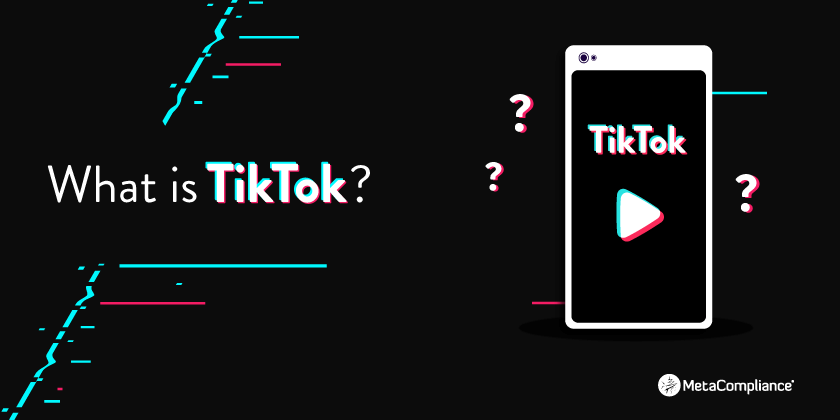The advertisement features a predominantly black background with the phrase "What is TikTok?" prominently displayed on the left. The text is set against a striking aqua and red graphic that resembles a slanted street—beginning at the bottom left corner and rising to about a quarter into the top right. A smartphone is showcased at the center of the image, displaying the TikTok app screen which is primarily dark with an arrow and question marks surrounding it, emphasizing the inquisitive nature of the ad. Below the phone, the ad credits "Meta Compliance" as the creator of the banner or page, though it leaves the viewer questioning the relationship between Meta Compliance and TikTok. The design is minimalistic, utilizing clean, straightforward text with subtle details that mimic TikTok's iconic color scheme—white text with aqua shading and pink or red accents.